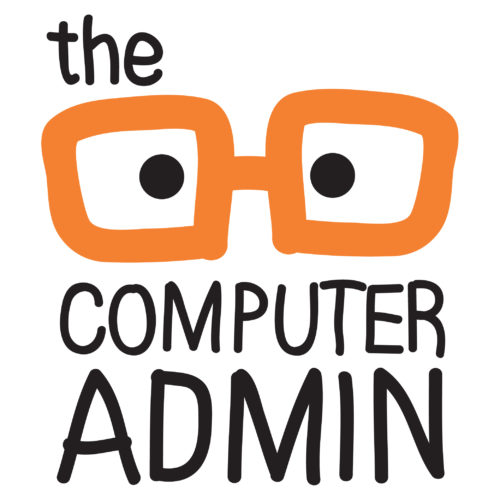The image is an illustration, likely created on a computer program like Microsoft Paint, featuring a design that could serve as a logo or icon for a YouTube channel or website. It presents a minimalist style with a pure white background and consists mainly of text and a drawing of glasses. The words "the", "computer", and "admin" are displayed in a large, bold black font. "The" is positioned at the top, "computer" in the middle, and "admin" at the bottom. In the center of the image between the text, there is a large depiction of glasses drawn with thick orange lines. Each lens contains a round, black eyeball-like dot towards the inner edges. The glasses, with their heavy orange outline and black details, draw significant attention amidst the otherwise stark and simple color palette of white, black, and orange.